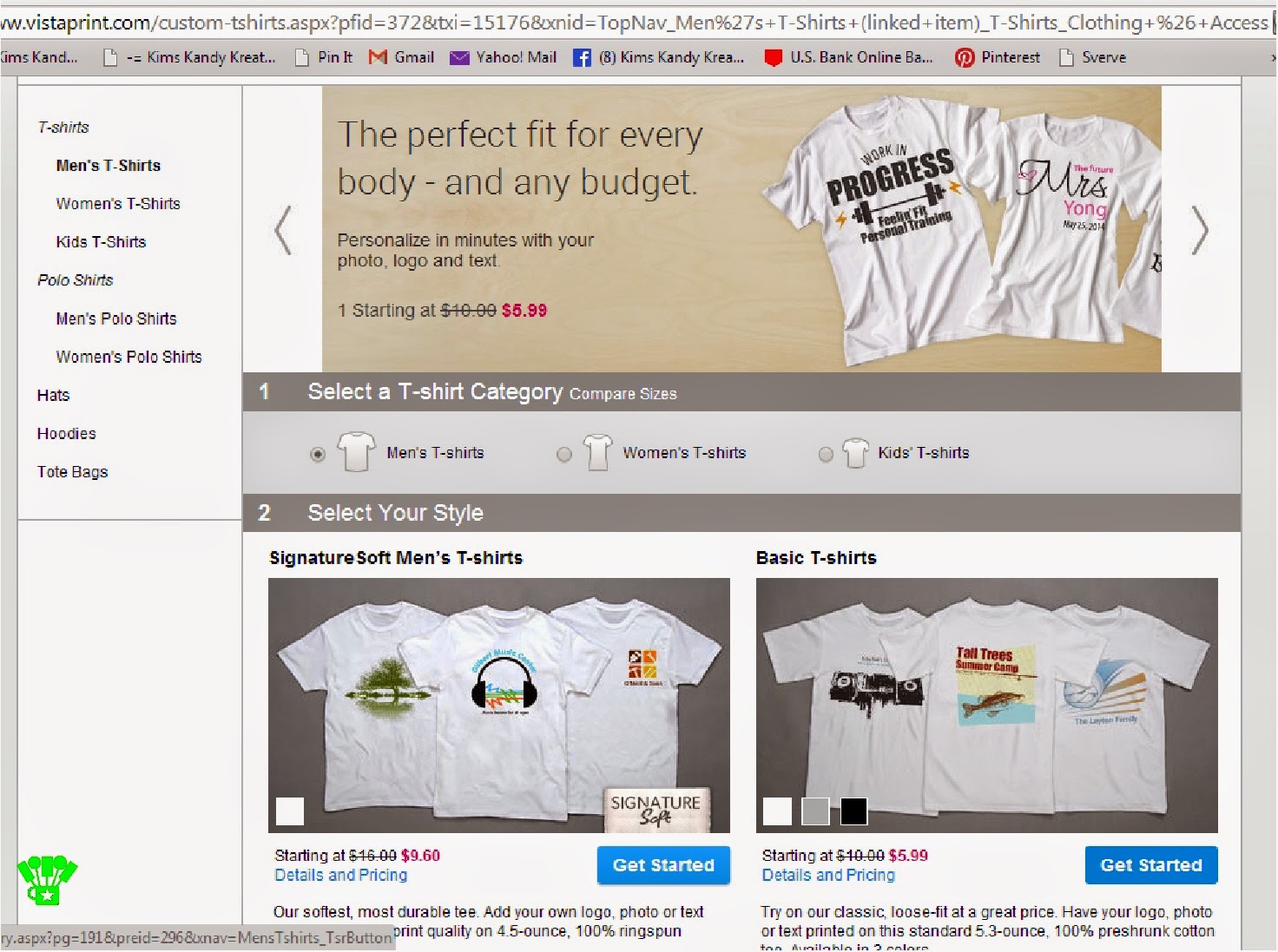This image features a screenshot of the Vistaprint website, specifically the section dedicated to designing custom t-shirts. At the top of the page, the Vistaprint logo is prominently displayed. The left sidebar lists various customizable apparel categories, including Men's T-shirts, Women's T-shirts, Kids' T-shirts, Polo Shirts, Hats, Hoodies, and Tote Bags. The sidebar also boasts a slogan: "The perfect fit for everybody on any budget."

Central to the image is a promotional banner encouraging users to "Personalize in minutes with your photo, logo, and text," with prices starting at $5.99. To the right, there are sample t-shirts displaying different fonts and design themes. Below the promotional banner, users are prompted to "Select a t-shirt by category," with options for Men's, Women's, or Kids' t-shirts.

Further down, the page is divided into sections. The first section, labeled "Select your style," showcases images of various t-shirts. Signature Soft Men's T-shirts are featured on the left, priced at $9.60. To the right, Basic T-shirts are displayed, starting at $5.99. Each pricing option has an adjacent clickable text link that says "Get started," inviting users to begin their custom t-shirt design process.